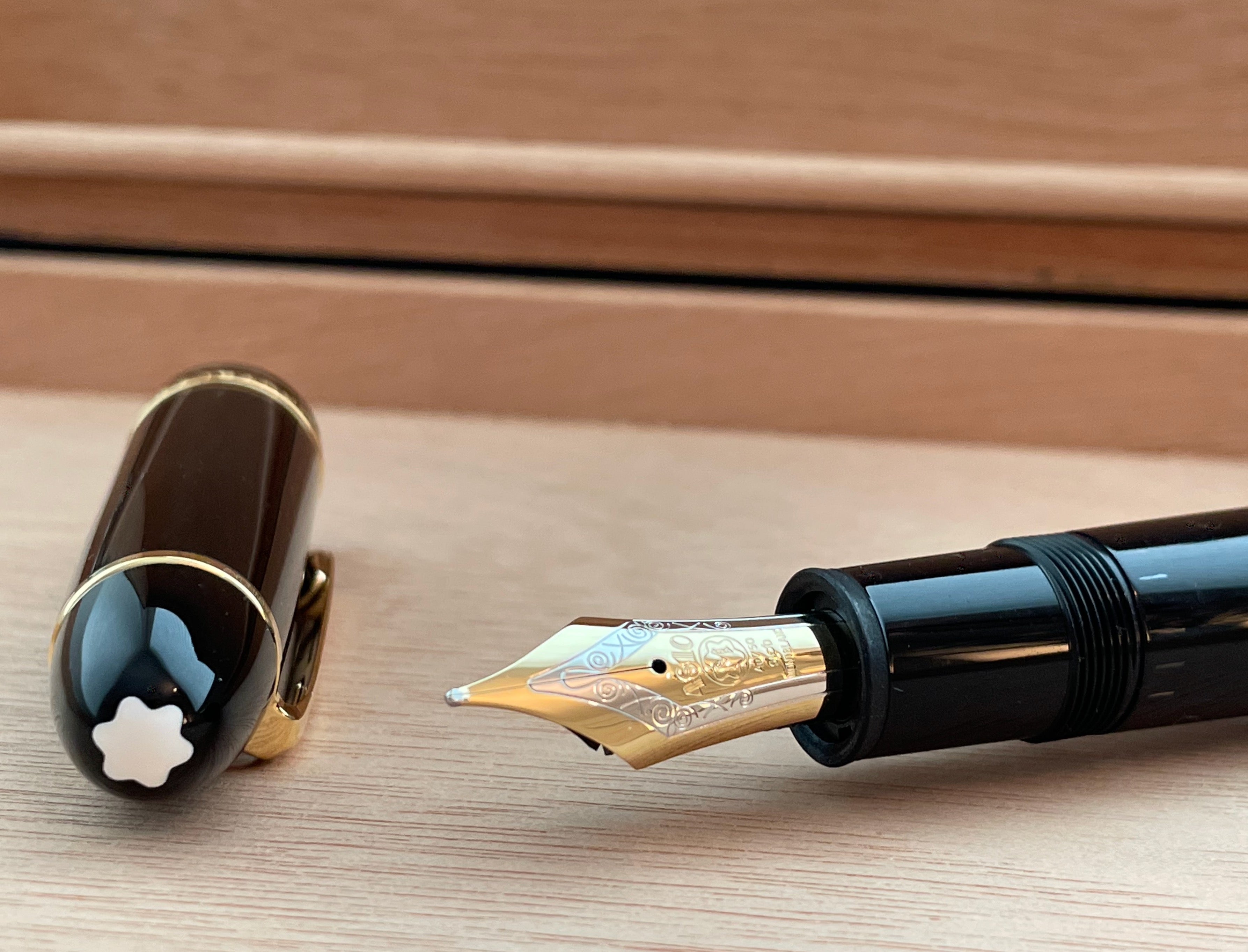This image is taken indoors, featuring a setting where the walls and surface are made of light-colored wood, creating an overall light brown background. In the foreground, there is a wooden surface with a noticeable wood grain texture. Resting on this surface are several shiny black fountain pens, which stand out due to their glossy finish. Each pen features a gold-colored, intricately designed tip that is quite pointed. The caps of the pens are removed, revealing thick black barrels adorned with a distinctive white star or flower petal shape on the end. Additionally, there's a gold clip on the caps. The overall scene is bathed in a soft, yellow light, accentuating the elegant and classical appearance of the fountain pens.